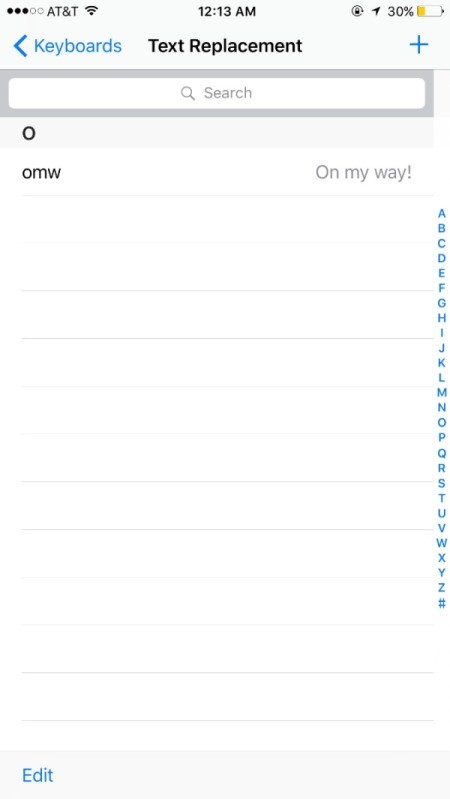This screenshot displays the "Keyboards" settings on an Apple iPhone, specifically focusing on the "Text Replacement" feature. This feature allows users to create shortcuts for commonly used phrases or words, enhancing typing efficiency. For instance, the user has programmed the letter "O" to automatically expand into "OMW," which stands for "on my way," whenever they type "O" in any text field. This personalized shortcut enables quicker communication by reducing the need to type the full phrase.

The text replacement options can be customized for any letter from A to Z and even include special characters such as the pound symbol (#), allowing for a variety of shortcuts tailored to individual needs. Currently, "O" is the only configured shortcut displayed in this screenshot, though the user may opt to add more shortcuts over time.

At the bottom of the screen, there is an "Edit" button, permitting users to modify or delete existing shortcuts. Additionally, a blue "+" button is located at the top right corner, which provides a straightforward way to add new text replacements. This functionality, found under the "Keyboards" section, is designed to streamline typing tasks and make the iPhone experience more efficient and user-friendly.